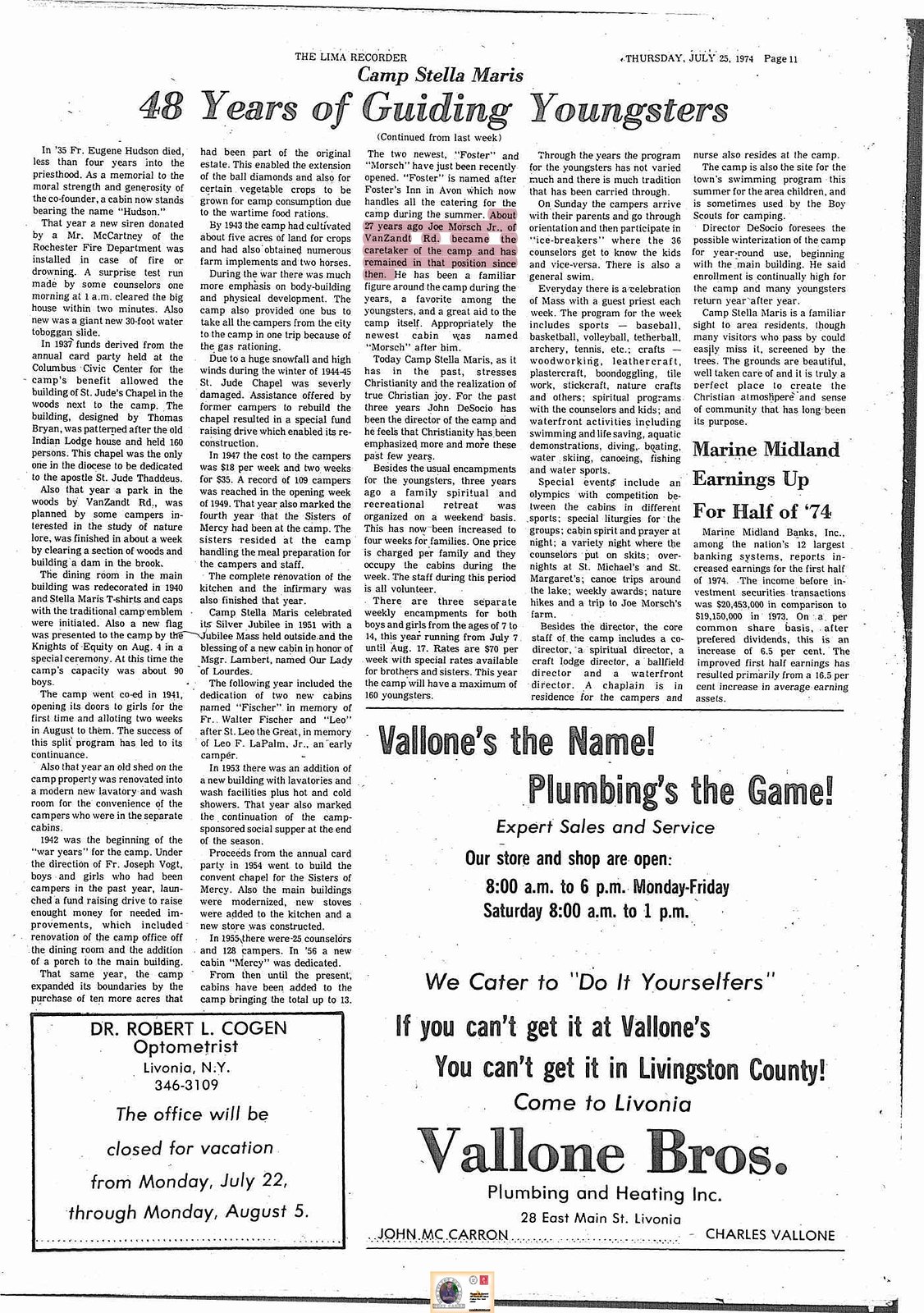This is an image of a vintage newspaper clipping from "The Lima Reporter Recorder," dated Thursday, July ?, 1974. The headline "48 Years of Guiding Youngsters" sits prominently at the top. 

The article commemorates the nearly five decades of Camp Stella Maris' influence on young people. A notable mention within the article is the tragic story of Fr. Eugene Hudson, who died within four years of his priesthood; a cabin named Hudson was erected in his honor. That year, the camp also benefited from a donated siren from Mr. McCartney of the Rochester Fire Department, tested successfully by counselors at 1 a.m. Moreover, 1937 saw the completion of St. Jude's Chapel, funded by the camp's annual card party held at the Columbus Civic Center, along with the installation of a 30-foot water toboggan slide.

The newspaper also includes an advertisement for Valone Brothers Plumbing and Heating, boasting their expert sales and service, open Monday through Friday from 8 a.m. to 6 p.m., and Saturdays from 8 a.m. to 1 p.m., with a promise to cater to do-it-yourselfers. Another advertisement by Dr. Robert L. Cogan, an optometrist in Livonia, New York, notes that his office would be closed for vacation from July 22nd to August 5th.

Lastly, the paper includes economic news with an article titled "Marine Midland Earnings Up Half of '74," indicating a promising financial update for that period. This rich fragment provides a snapshot of historical events and local business life from nearly five decades ago.